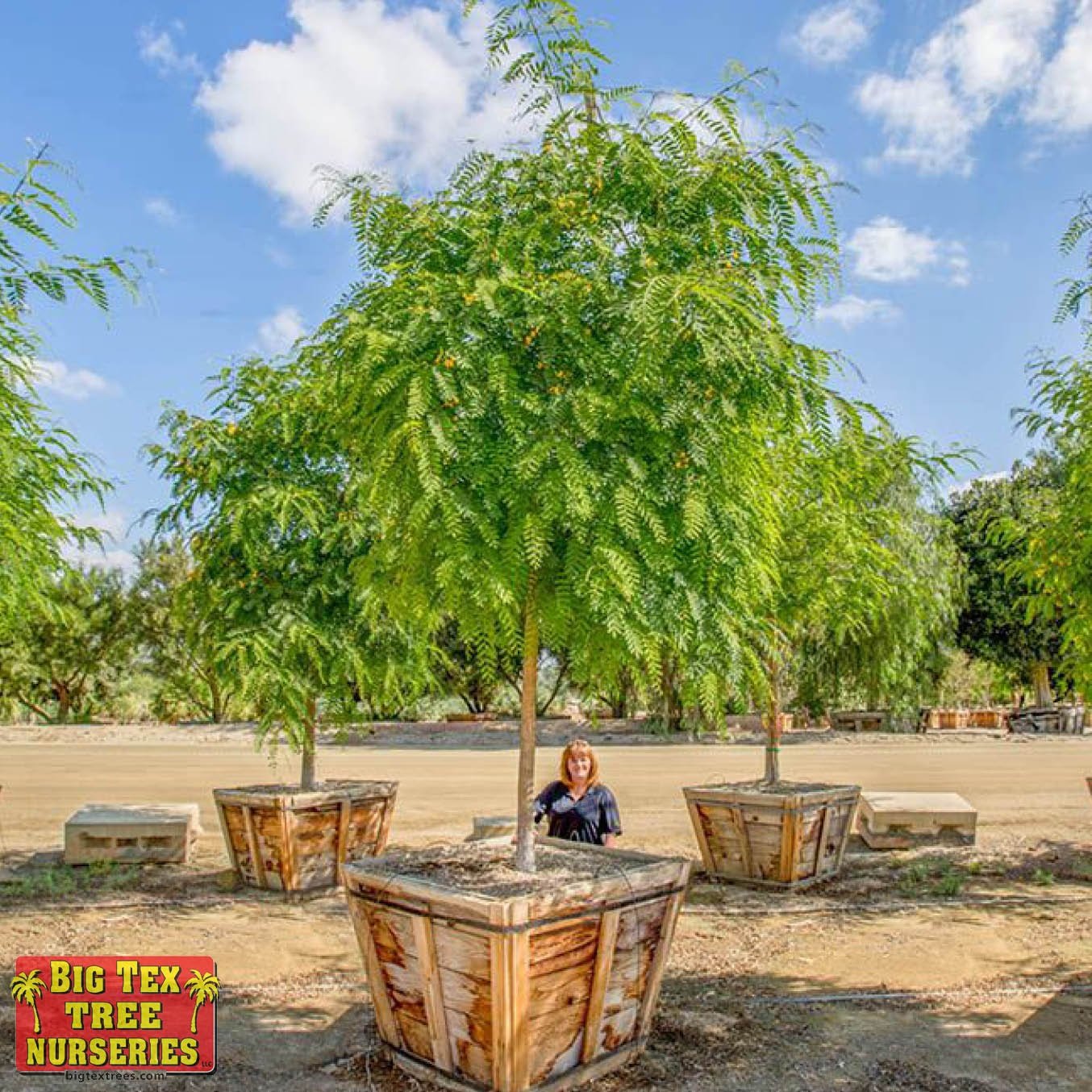In this color photograph, a Caucasian woman with long red hair stands behind a central wooden planter box, which contains a medium-sized tree with lush green leaves. She is dressed in dark blue clothing. The planter boxes, constructed from wooden planks, have a tapered design at the bottom and are filled with brown earth. Additional planter boxes with similar trees flank her on either side. The scene captures a tree nursery's organized layout, with more trees planted in the ground visible in the background under a vibrant blue sky dotted with white, fluffy clouds. In the bottom left corner of the image, a red rectangle with rounded corners displays the yellow text "Big Tex Tree Nurseries" along with small logos of palm trees. Below this, the website "trees.com" is prominently displayed. The ground is covered in brown sand, providing a natural backdrop to the serene and well-maintained nursery setting.